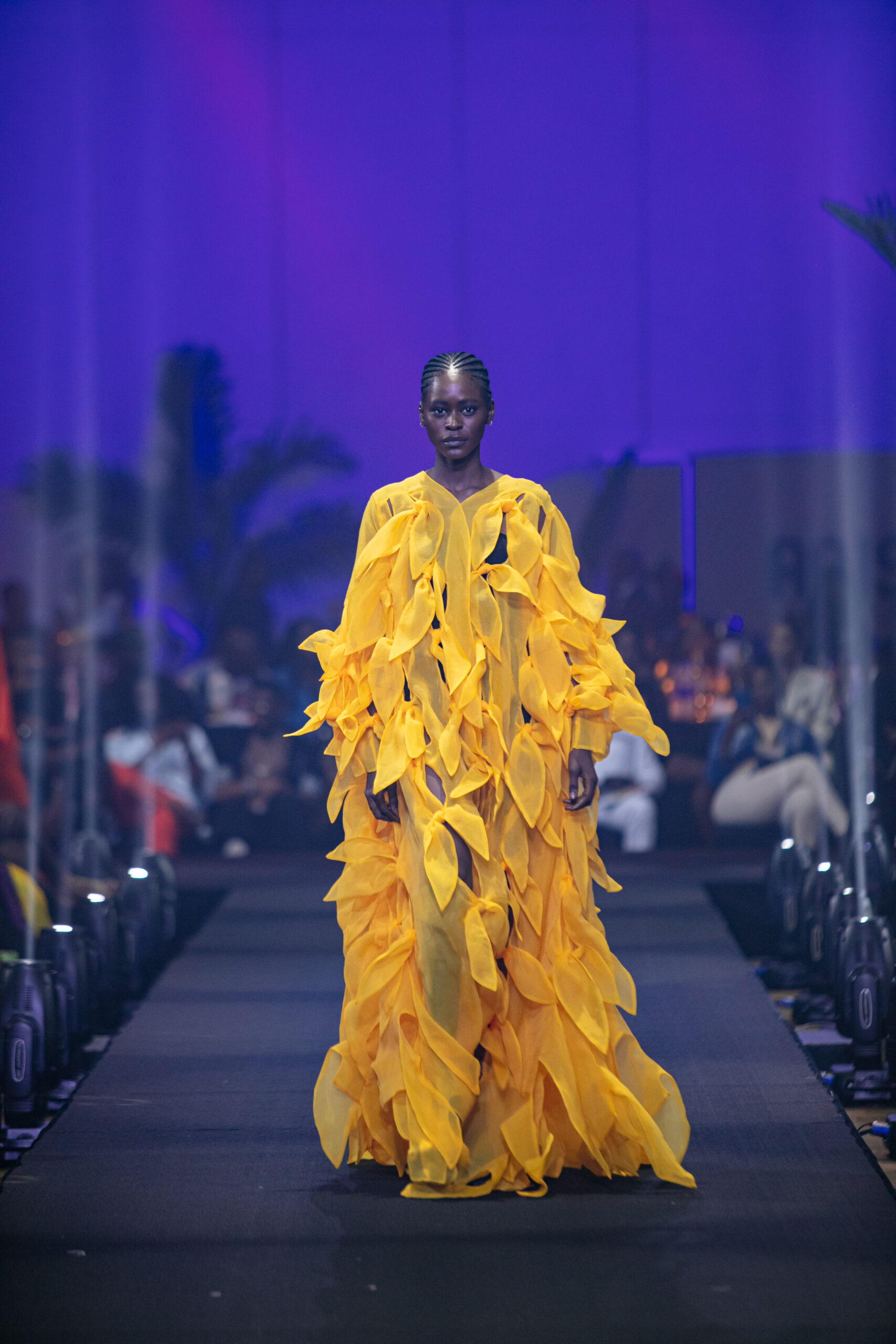In this image, a model is confidently walking down a black carpet runway at a fashion show. The runway is flanked by eight powerful spotlights, four on each side, shooting beams of light upwards into the air, creating a striking visual effect. The backdrop is a dark purple hue, adorned with the silhouette of a palm tree, adding to the ambiance of the scene. Behind the model, slightly out of focus, is an audience seated in rows, attentively watching. The model, with a darker complexion, has her hair styled in intricate cornrows and is wearing statement earrings. Her outfit is a bright yellow, flowy dress that stands out vividly against her skin tone. The dress features a sheer leaf or feather-like pattern throughout, and is designed with ruffled sides and knee cutouts, adding dynamic elements to her look.